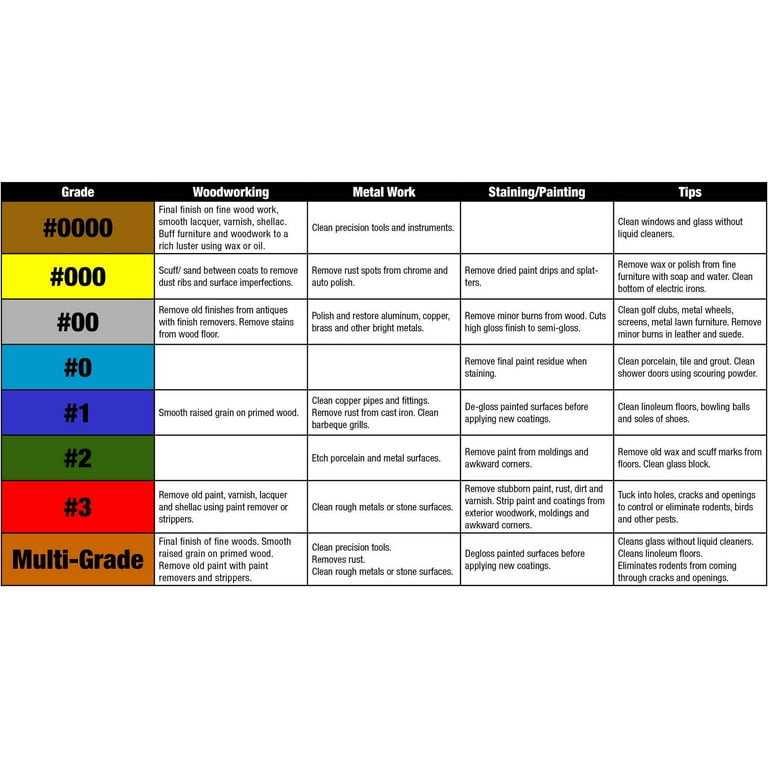This image shows an informational sheet for paint, organized into a grid with five columns and nine rows set within a horizontal rectangle. The top row features a black, thin border with white text headings: Grade, Woodworking, Metalwork, Staining & Painting, and Tips. Below the Grade column, there are eight rectangular cells, each colored differently, labeled as follows: #0000, #000, #00, #0, #1, #2, #3, and Multi-Grade. The remaining columns provide detailed information related to each grade, focusing on specific tasks. For example, the Metalwork column includes tasks such as cleaning precision tools, removing rust spots from chrome, auto-polishing, and restoring metals like aluminum, copper, and brass. Similarly, the Woodworking, Staining & Painting, and Tips columns offer corresponding advice and instructions, making the sheet a comprehensive guide for various paint-related activities.